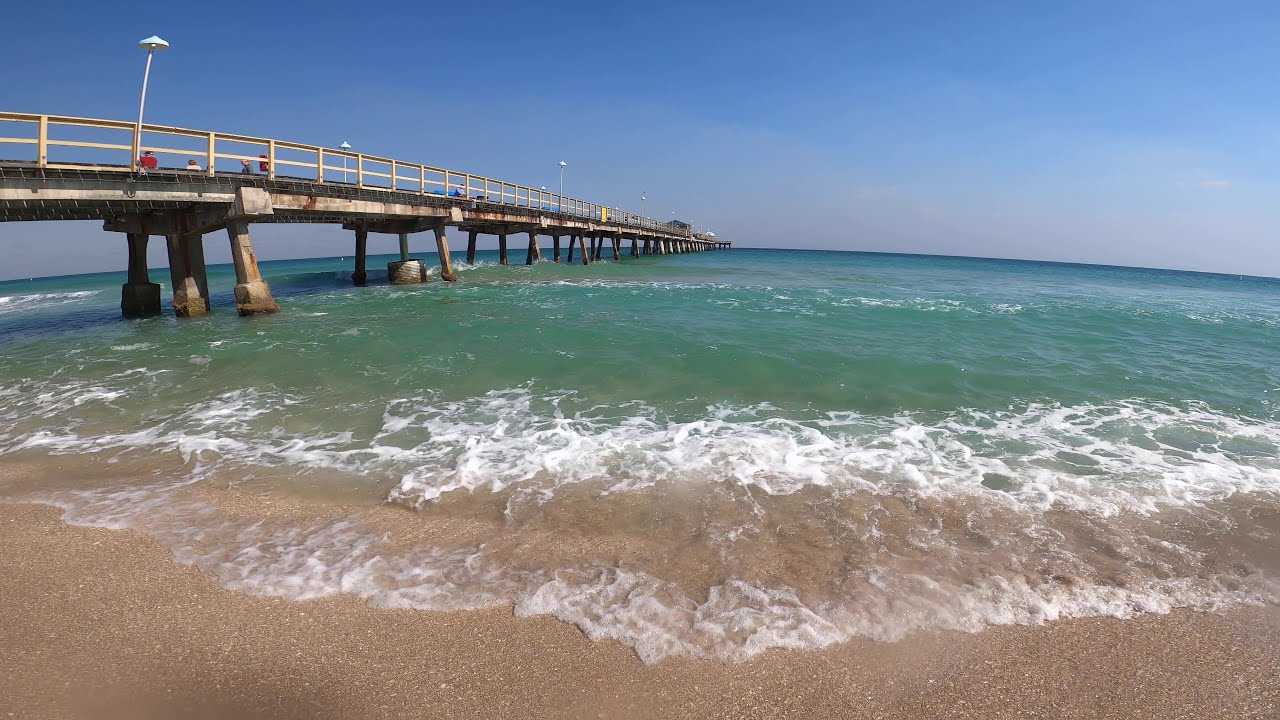A horizontal, rectangular photograph captures a tranquil beach scene with vivid detail. The foreground features a sandy beach where small waves, foamy and white, crash gently against the shore. The water showcases a gradient, transitioning from a clear, brownish hue near the sand to a beautiful aqua and then green, eventually blending into a deep blue further in the distance. The sky above is mostly clear, adorned with occasional clouds and a bright, inviting blue.

On the left side of the image, an old, lengthy pier—or possibly a bridge—extends far out into the ocean. The pier’s supporting structures, likely once white, are now coated with rust, adding character and history to the scene. There are streetlights atop the pier, and people can be seen walking or sitting along its length. At the end of the pier, there's a distant structure that could be a restaurant or a rest area, inviting visitors for a closer look. The pier spans at least a mile, merging with the horizon where the endless ocean meets the sky. The entire scene is bathed in natural light, encapsulating the serene beauty of the beach.